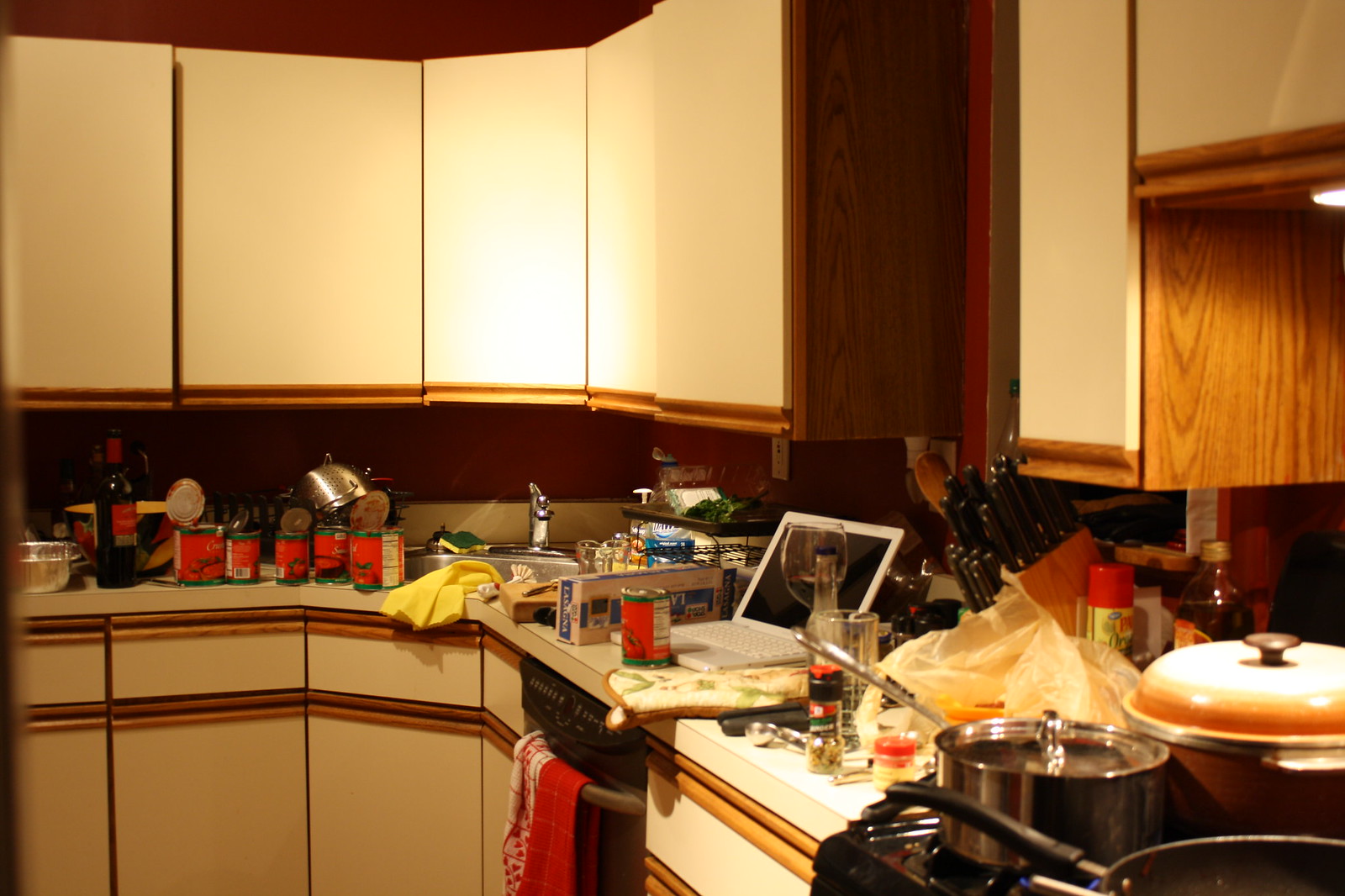The image depicts a cluttered kitchen with a mix of white and brown cabinetry. The upper cupboards are all white and feature a lighter brown line near the bottom, presumably for opening. The lower floor cupboards have rectangular shelves and white doors, accentuated by two brown lines running horizontally for easy access to both the top and bottom sections.

At the center of the kitchen, there is a table with a mix of items: a black wine bottle, a yellow container behind it, and five cans of food with orange labels. A silver pot and a pan are situated at the back of the table. In the corner, there is a sink with a yellow dish cloth draped over it and a wash sponge placed on top. Nearby, there is a brown chopping board and some boxes, one of which holds another orange-labeled can of food. There is also an open white PC.

Underneath the counter is an oven with an orange rack atop it. Beside it, several spices, a bottle, a knife holder, and another cupboard are visible. Finally, the stove, equipped with four pots, completes the scene.

Overall, the kitchen appears highly cluttered, with a variety of items dispersed across the counters and table, suggesting recent activity or an ongoing culinary project.